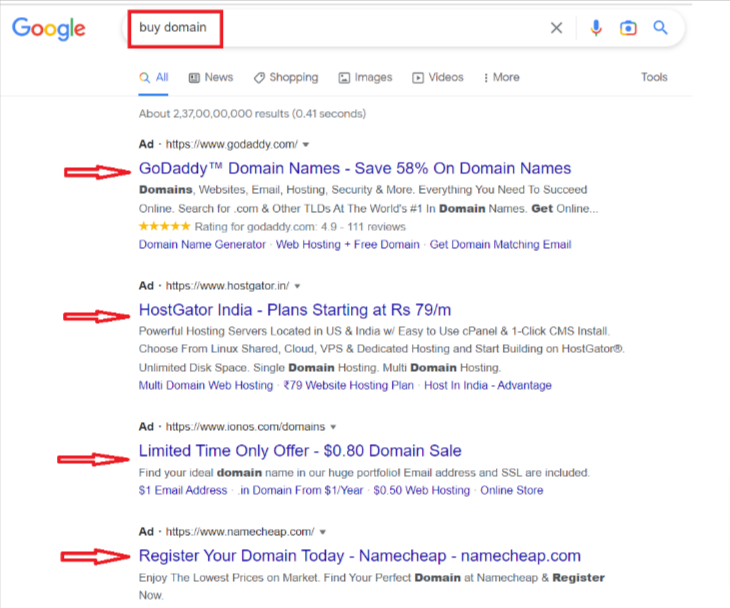The image features a clean white background with very light blue lines, creating a minimalist design. At the top, there are two small light blue lines followed by the iconic Google logo, displaying the letters in blue, red, yellow, and green. Below the logo sits a small red box with a white interior that reads "by domain" in gray letters.

Next to this box is a row of icons: an 'X', a microphone, a screen, and a magnifying glass, followed by a circle containing a small square with a circle inside it. Underneath these icons is a blue underlined text, highlighting different categories such as "News," "Shopping," "Images," "Videos," and "More," with "Tools" appearing at the very end.

The image also includes several advertisements, each marked by a red arrow pointing to the right. The first ad promotes GoDaddy with a message that says, "GoDaddy domain name, save 58% on domain names." The second advertisement, marked again by a red arrow, is for HostGator India, stating, "Plans starting at ₹79/month." The third ad features a limited-time offer, "80-cent domain sale." Finally, the fourth advertisement encourages users to "Register your domain today" at Namecheap, with the URL "namecheap.com" indicated.

This image effectively captures a snapshot of a Google search page with an array of advertisements for domain registration services.